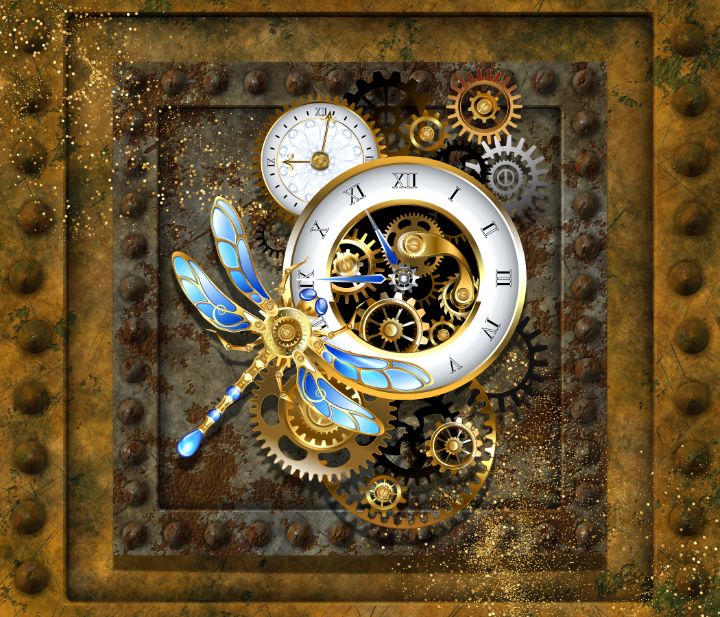The image depicts the intricate workings of a clock, set against a luxurious backdrop composed of multiple nested frames. The outer frame is gold, adorned with darker gold knobs or tacks around the edges. Within this is another frame of similar gold, and then an inner frame of dark gray and brown with more of the same knobs or tacks. Central to the image is a clock reading approximately 9:03, featuring a beautiful watch face ringed in gold with a light blue border. The clock face displays Roman numerals and is graced by a stunning dragonfly in shades of blue and yellow, perched delicately on the clock. Behind this foreground, a complex array of dials and gears typical of a clock’s interior mechanics are visible, adding to the elaborate depth and detail of the scene. The entire composition gives a sense of timeless elegance, with hints of golden sparkles and a slightly shiny, though aged, appearance.